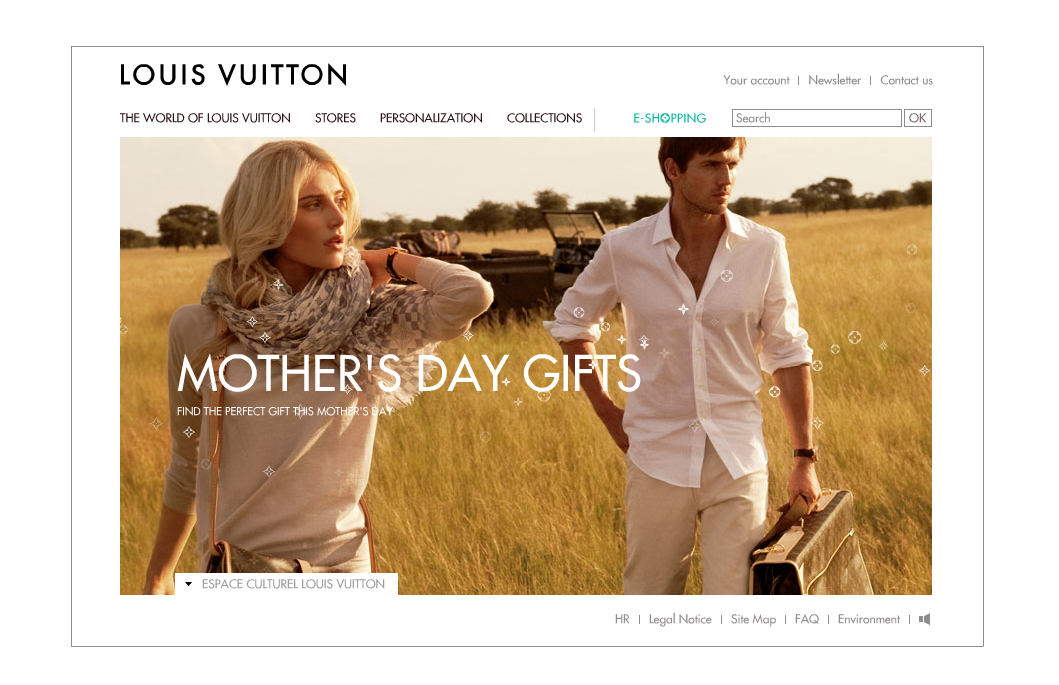The image depicts the Louis Vuitton homepage. Prominently displayed at the top left is the Louis Vuitton logo in black, set against a pristine white background. Beneath the logo, several navigation options in brown include "The World of Louis Vuitton," "Stores," "Personalization," and "Collections." Below these, a teal-colored section labeled "eShopping" introduces a thematic shift, followed by a search bar on the far right, which includes an "OK" button. 

Above the search bar, links are arranged horizontally for easy access to "Your Account," "Newsletter," and "Contact Us," each separated by small dividers. Dominating the central area is a title in large, stylish text that reads "Mother's Day Gifts," along with a tagline, "Find the perfect gift this Mother's Day."

Situated below the text is a striking photograph featuring a sophisticated woman, possibly representing a mother, and a young man standing behind her with a Louis Vuitton bag. Both exude a luxurious ambiance, further heightened by the exotic backdrop that resembles the Sahara desert or an African savanna. The duo appears to have just disembarked from a Jeep, embodying the epitome of elegance and style amid rugged surroundings, showcasing the allure of Louis Vuitton's exclusive Mother's Day offerings.